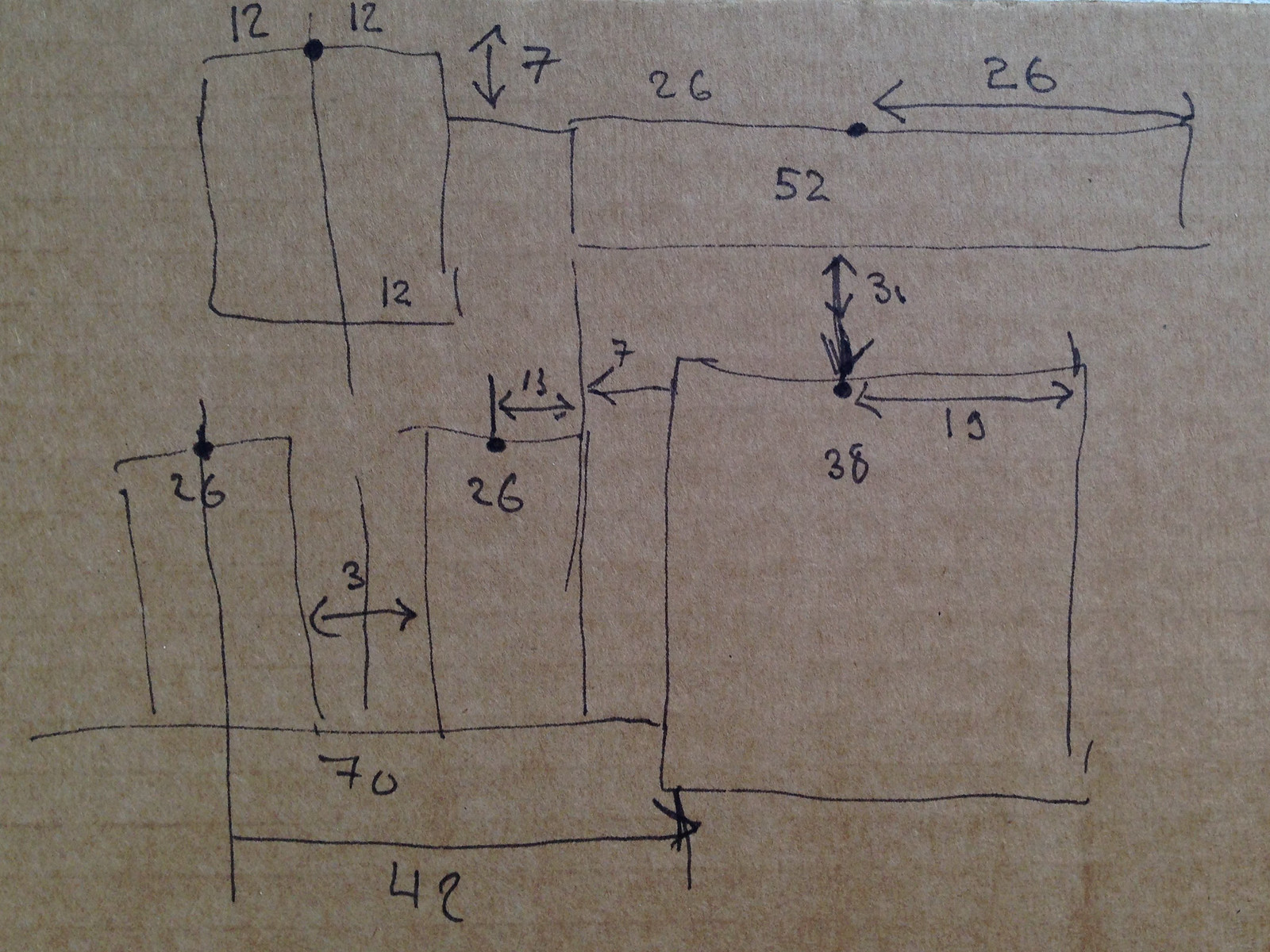The image features a detailed architectural or engineering diagram. In the top left corner, there is a square marked with the number 12 at the midpoint of its top side. A dot is placed at the midpoint with the number 12 repeated. At the bottom right of the square, the number 12 is labeled again. A line intersects this square vertically from the top dot down to the bottom side.

This square is connected by a line to a long rectangle. This connecting line is marked with an arrow pointing vertically, labeled with the number 7, indicating a 7-foot difference between the 12-foot square and the adjacent piece. The rectangle itself contains the numbers 26 at both ends, divided by a dot, summing up to a total of 52 within the rectangle.

Below this rectangle is another vertical arrow with the number 31. This connects to a square beneath it marked with an arrowed line pointing horizontally. This arrowed line leads to a dot near the center, labeled with the number 38.

Adjacent to this setup are two additional smaller rectangles, each marked with the number 26. At the bottom of the diagram is a long rectangle labeled with the number 70.